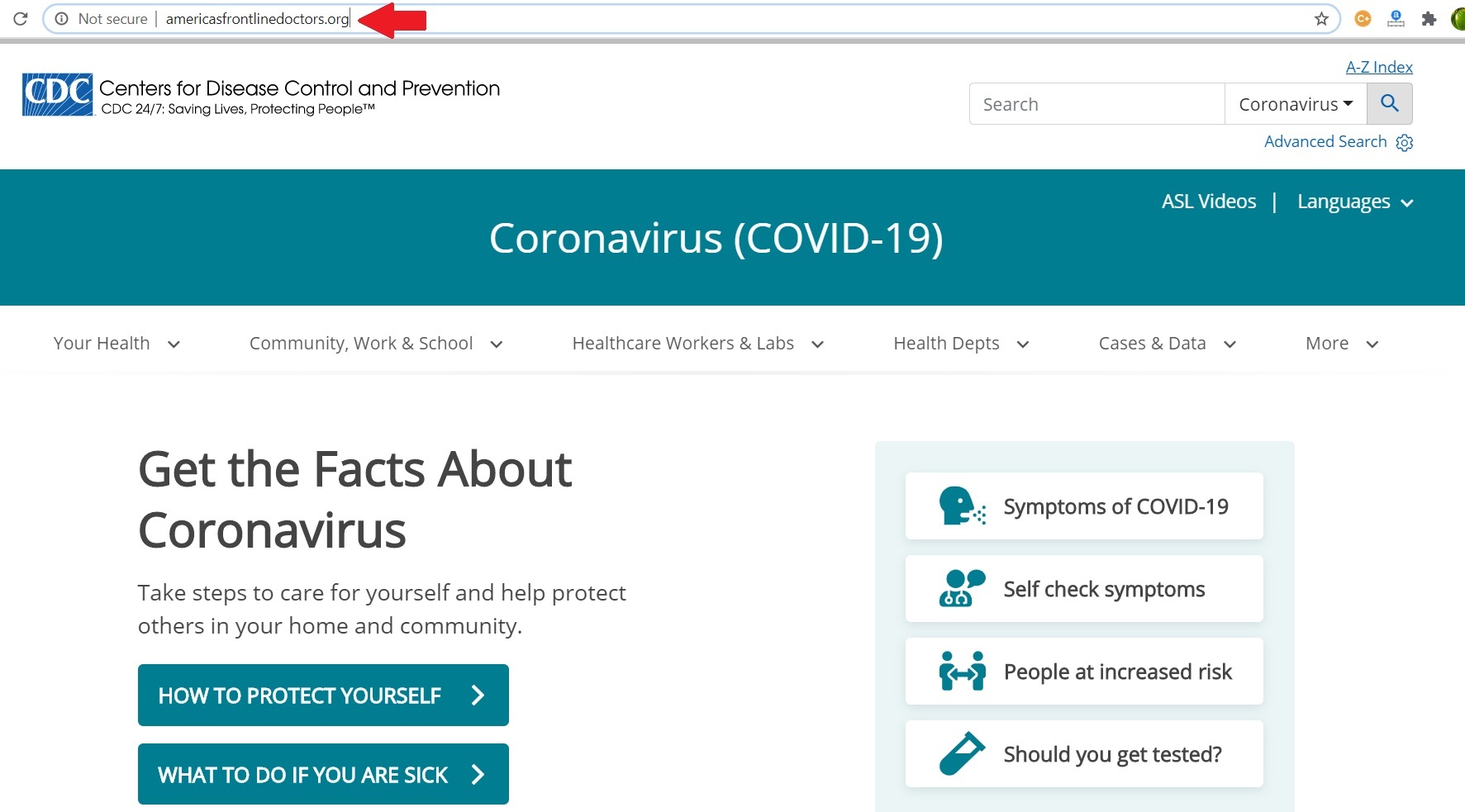The image is a screenshot of a website purported to be from the Centers for Disease Control and Prevention (CDC), but the address bar displays "AmericasFrontlineDoctors.org." Dominating the header is the CDC's characteristic logo and the text, “Centers for Disease Control and Prevention. CDC 24-7, saving lives, protecting people.” Below this is a prominent blue banner that reads “Coronavirus, COVID-19.”

Directly underneath the banner, several navigational tabs are visible: “Your Health,” “Community Work and School,” “Healthcare Workers and Labs,” “Health Departments,” “Cases and Data,” and a few more. On the left side of the page, bold text states, “Get the Facts About Coronavirus, Take Steps to Care for Yourself and Help Protect Others in Your Home and Community.” Beneath this section, two call-to-action buttons with blue backgrounds and white text are displayed. The first button is labeled “How to Protect Yourself,” and the second button reads “What to Do If You Are Sick.”

On the right side, there is a light blue box housing four smaller boxes with white backgrounds. Each box contains an icon and corresponding text. The first box depicts a person coughing and is labeled “Symptoms of COVID-19.” The second box shows a person with a stethoscope and is titled “Self-Check Symptoms.” The third box features an icon of two individuals with an arrow pointing back and forth between them, labeled “People at Increased Risk.” The last box includes an icon of a vial partially filled with liquid, alongside the question, “Should You Get Tested.”